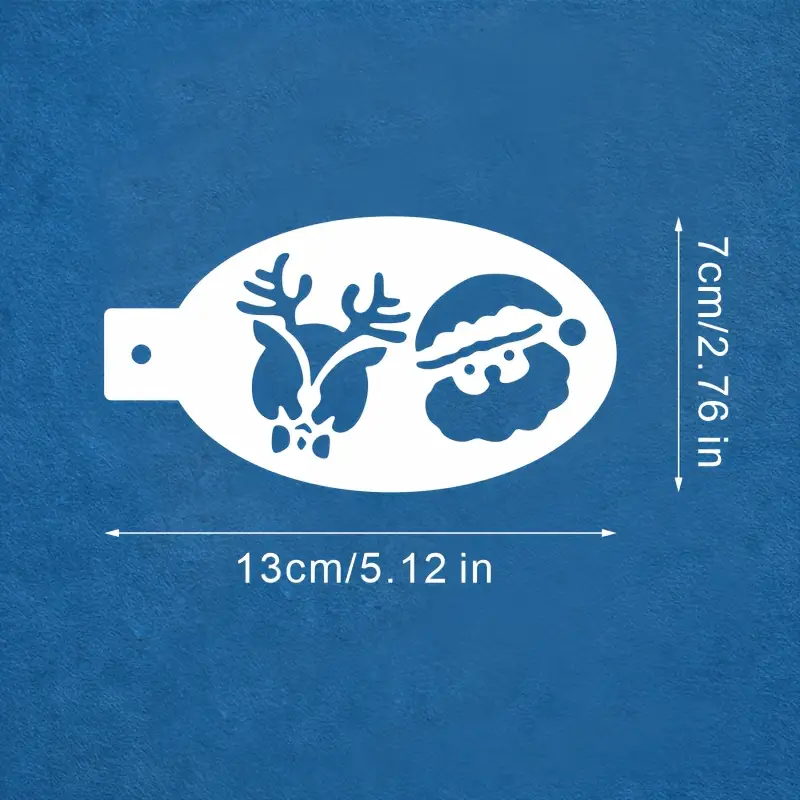The image depicts a detailed Christmastime design with a festive theme, set against a navy blue, textured background resembling ocean water. Central to the image is a white, horizontally-placed oval shape resembling the head of a spoon. This oval contains blue, cartoon-style illustrations: on the left, a reindeer's head complete with antlers and a bow tie, and on the right, Santa Claus's head with his iconic hat, both featuring prominent negative white spaces for facial details and accessories. The design appears like a logo, sticker, or holiday card, enhanced by precise measurements indicated around it – 7 cm (2.76 inches) tall noted on the right side, and 13 cm (5.12 inches) wide along the bottom edge. A rectangular tag portion extends from the left side of the oval, and there's a circular cutout on the left side of the rectangular section.